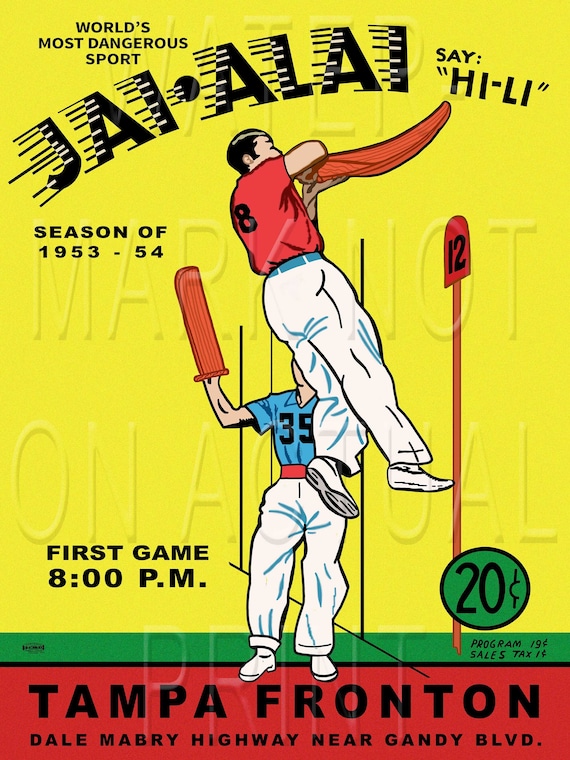This image showcases a vintage poster advertising the sport of Jai Alai, heralded as the "World's Most Dangerous Sport." Dominating the poster is the highly stylized title "Hialeahe" in a dynamic font with black stripes streaming from each letter, emphasizing high speed and excitement. Adjacent to this, the text assists with pronunciation: "Say, Hi, Lie, H-I-L-E-I." Below, details of the event are listed: "Season of 1953-1954" and "First Game, 8pm." In the bottom right corner, a green circle announces the entry fee: "$0.20," and further below, program costs at "$0.19" with an additional "$0.01" for sales tax are noted. A striking red banner at the bottom provides the event location in black text: "Tampa-Fronton-Dale-Mabry-Highway-Near-Gandee-Boulevard."

The background is predominantly yellow, enhancing the vibrancy of the poster. Set against this backdrop are two Jai Alai players in action. The foreground features a player, mid-air, wearing a red shirt with the number 8, and white trousers and shoes. He is captured in a dynamic pose, his cesta—a curved basket used to catch and throw the ball—held supported by both hands. Behind him, a second player in a blue shirt with the number 35, white pants, a red belt, and white shoes, stands grounded in anticipation, his cesta held upright in his right hand. The scene is set in front of a series of lines marked by a pole displaying the number 12, indicating a part of the playing field. This poster, brimming with action and vintage charm, effectively conveys both the intensity of the sport and the specific event details in a nostalgic nod to the 1950s.